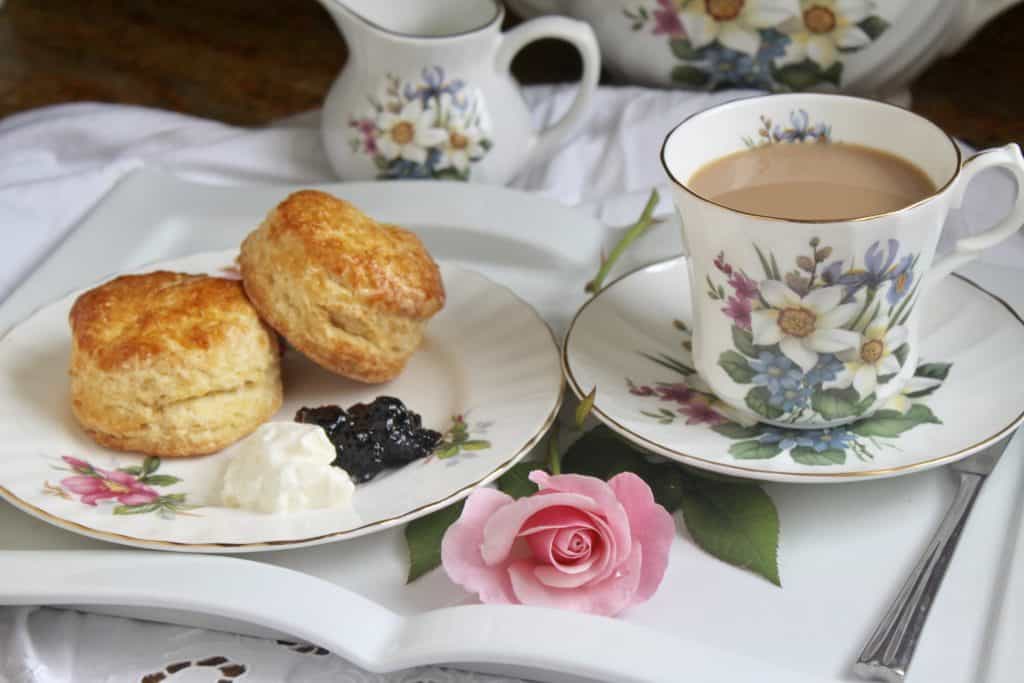This photograph captures an elegant breakfast or brunch setting characterized by a traditional English tea service. Central to the image is a delicate floral teacup filled with brown milk tea, resting on a matching saucer. This saucer partially covers a silver butter knife. To the left, a plate adorned with a pink floral print features two traditional English scones accompanied by clotted cream and jam. The setting is completed with a freshly cut pink carnation, adding a touch of natural beauty. In the background, a floral-patterned pitcher and part of a matching teapot are visible, suggesting the provision of cream or milk. All these elements are set atop a pristine white lace tablecloth, creating a cohesive and inviting scene that epitomizes a refined English tea experience.